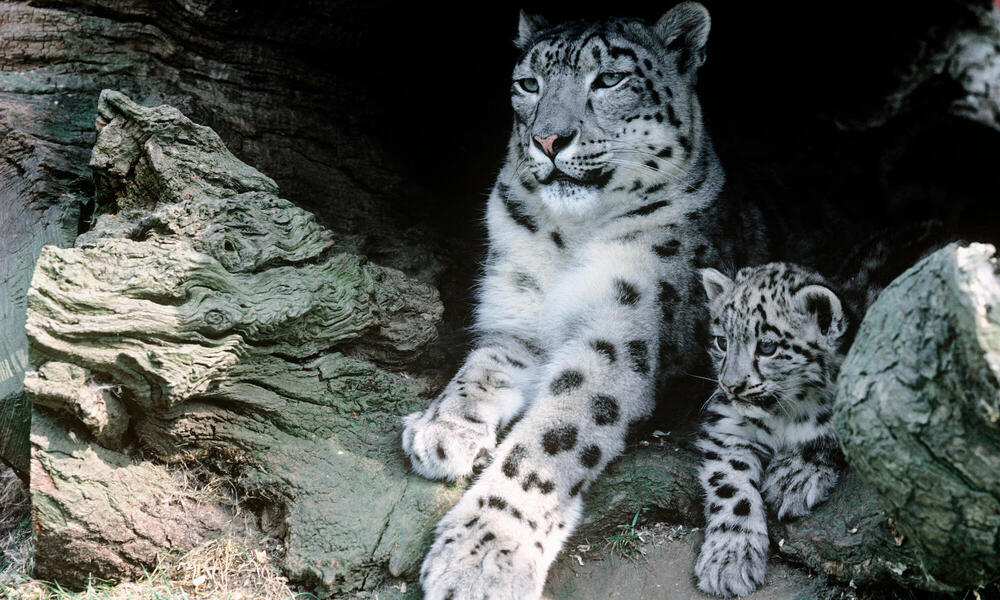This detailed photograph captures a pair of snow leopards, likely a mother and her young cub, positioned at the entrance of a dimly lit cave. Both majestic animals, marked with distinctive black spots on their pristine white fur, are lying down with one paw extended further than the other. The larger leopard is in the center, while the cub is positioned to her right, both gazing intently towards something outside the frame. Their eyes are a light color with hints of blue or blue-gray. The cave is surrounded by curvy rock formations, some appearing as petrified wood, along with deposits of green-colored igneous rock. The background fades into darkness, accentuating the intimate and serene setting of the snow leopards in their natural habitat.